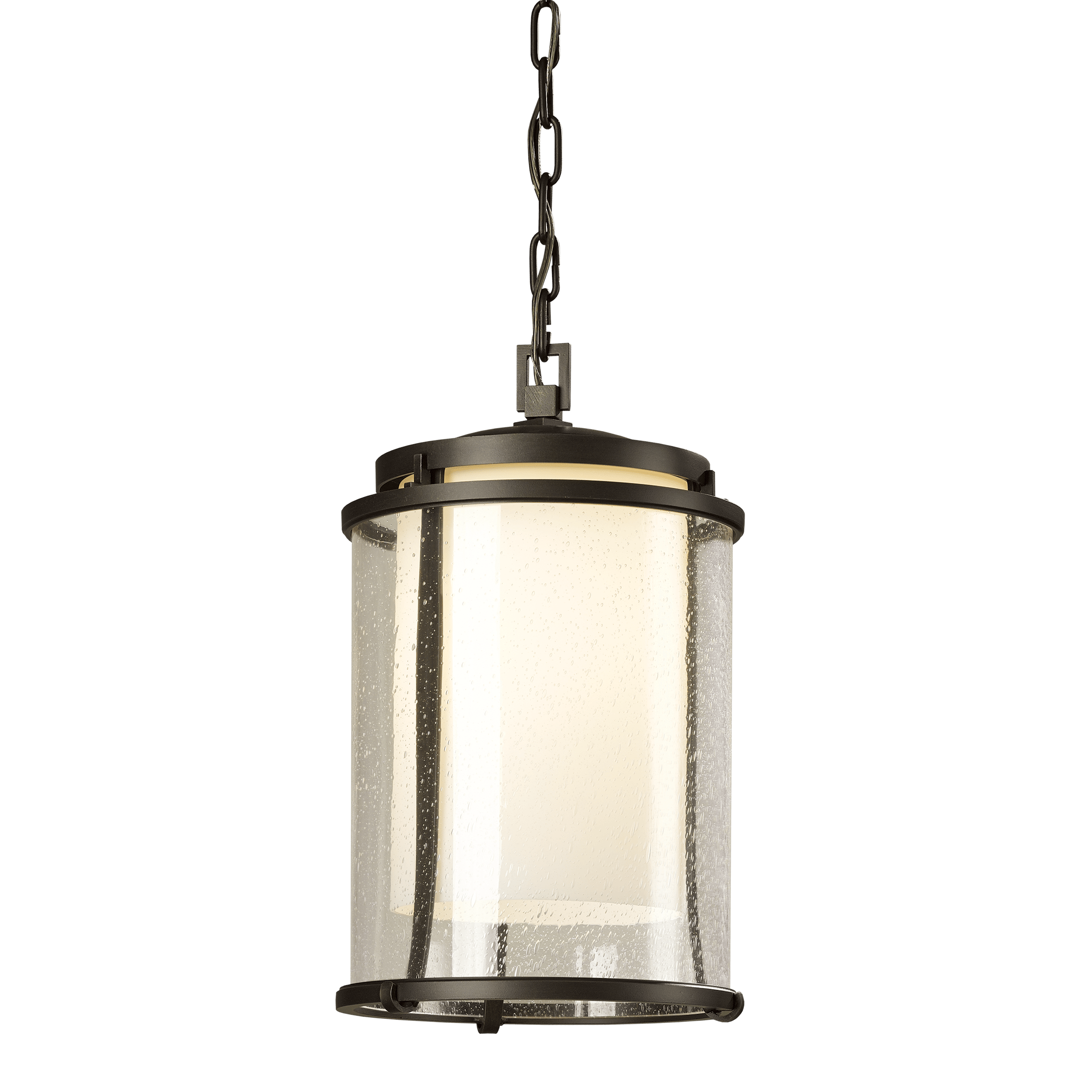This image features a modern pendant light, prominently displayed against a stark white background, emphasizing its design as a product image. The light hangs from a black chain, with an electrical wire neatly fed through the chain links. The lamp itself is a striking combination of black metal framing and a dual-cylinder glass design. The outer glass cylinder, appearing as if covered in water droplets, adds a visually appealing texture that contrasts with the smooth, opaque inner cylinder which hides the light source, emitting a soft yellow glow. The clear glass exterior and black accents give the lamp a sleek and contemporary look.